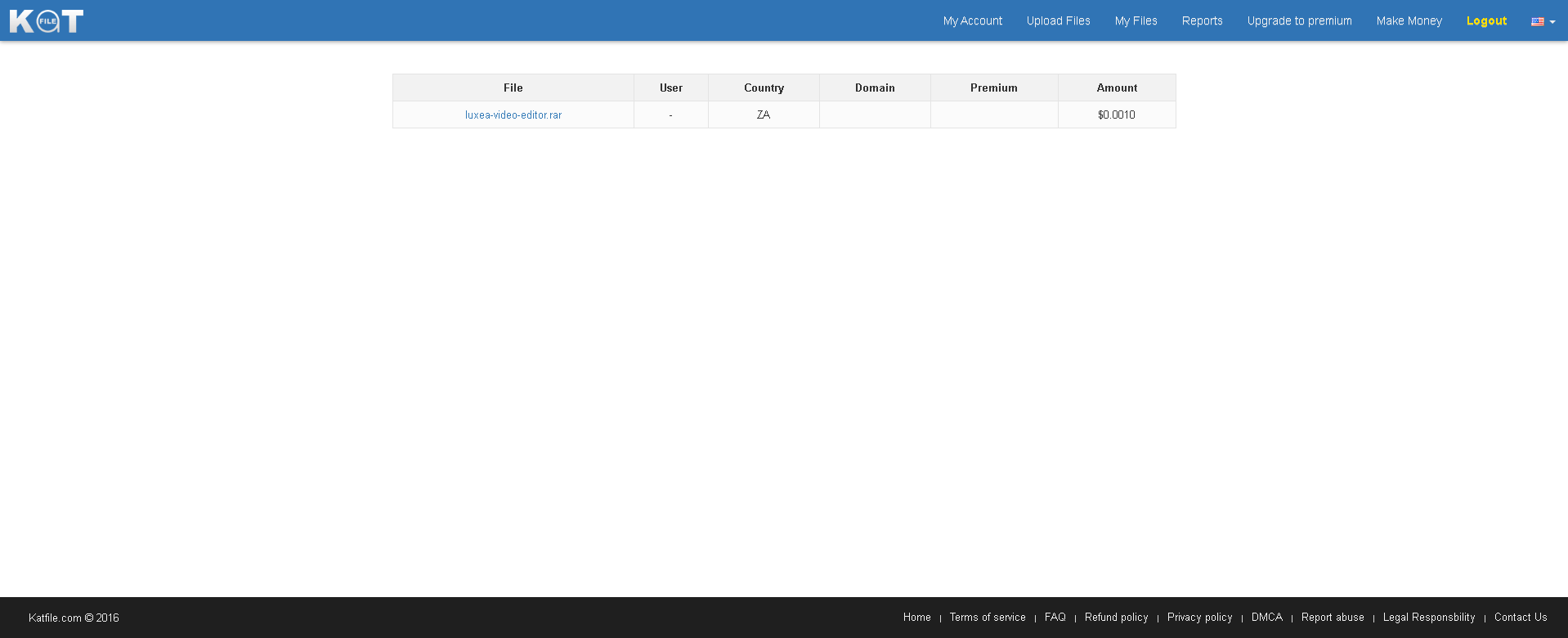This image is a screenshot of a web page with a simplistic and spacious design. The page, appearing in widescreen format, features a predominantly large, empty white space in its central area. At the top, there is a visually striking blue header, reminiscent of a horizontal bar, which serves as a backdrop for the site title and navigation options.

The title of the site is prominently displayed in the header, with the letters "K," "O" (represented as a white circle), and "T," all rendered in white. Adjacent to the title, on the far right side of the header, is a series of navigational buttons labeled: "My Account," "Upload Files," "My Files," "Reports," "Upgrade to Premium," "Move Money," and finally, "Logout," which is distinctively highlighted in yellow font.

In the extreme top-right corner, there is a small icon of the American flag, oriented to the right, adding a visual cue to the page's regional setting.

Centrally located on the page is a small window or table containing a single row of information. This table lists details such as a file name, country, and amount, yet the text is notably diminutive and challenging to discern, rendering it practically unreadable.